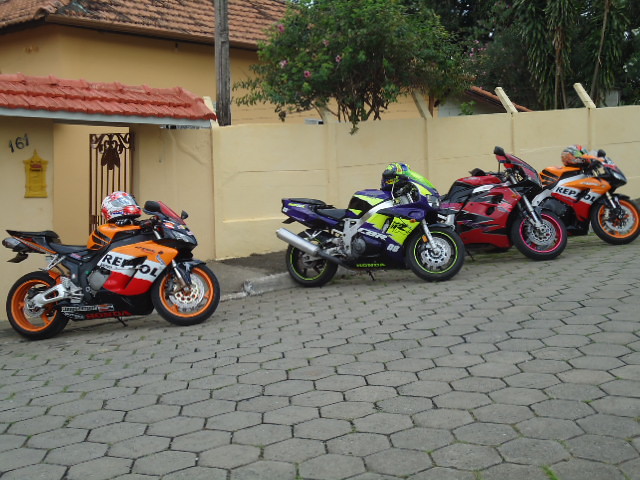The color photograph captures an exterior scene taken outside on a cloudy day with soft lighting, resulting in few shadows and a low-saturated hue. A line of sport-type motorcycles, featuring a variety of colors—orange, green, dark orange, yellow, purple, and red—are positioned against the curb on a gray cobblestone road composed of octagon pavers. The motorcycles tilt towards the center and to the right, with the orange bike on the far left slightly separated from the others. Each bike has a helmet positioned on the body behind the handlebars. They stand in front of a light yellow, stucco-style, Spanish-inspired building, indicative of architecture common in Mexico or Latin American countries. The building boasts a red tiled roof, a metal gate, and flowering trees behind the main fence area, creating a picturesque yet subdued backdrop for the vibrant motorcycles lined up below.